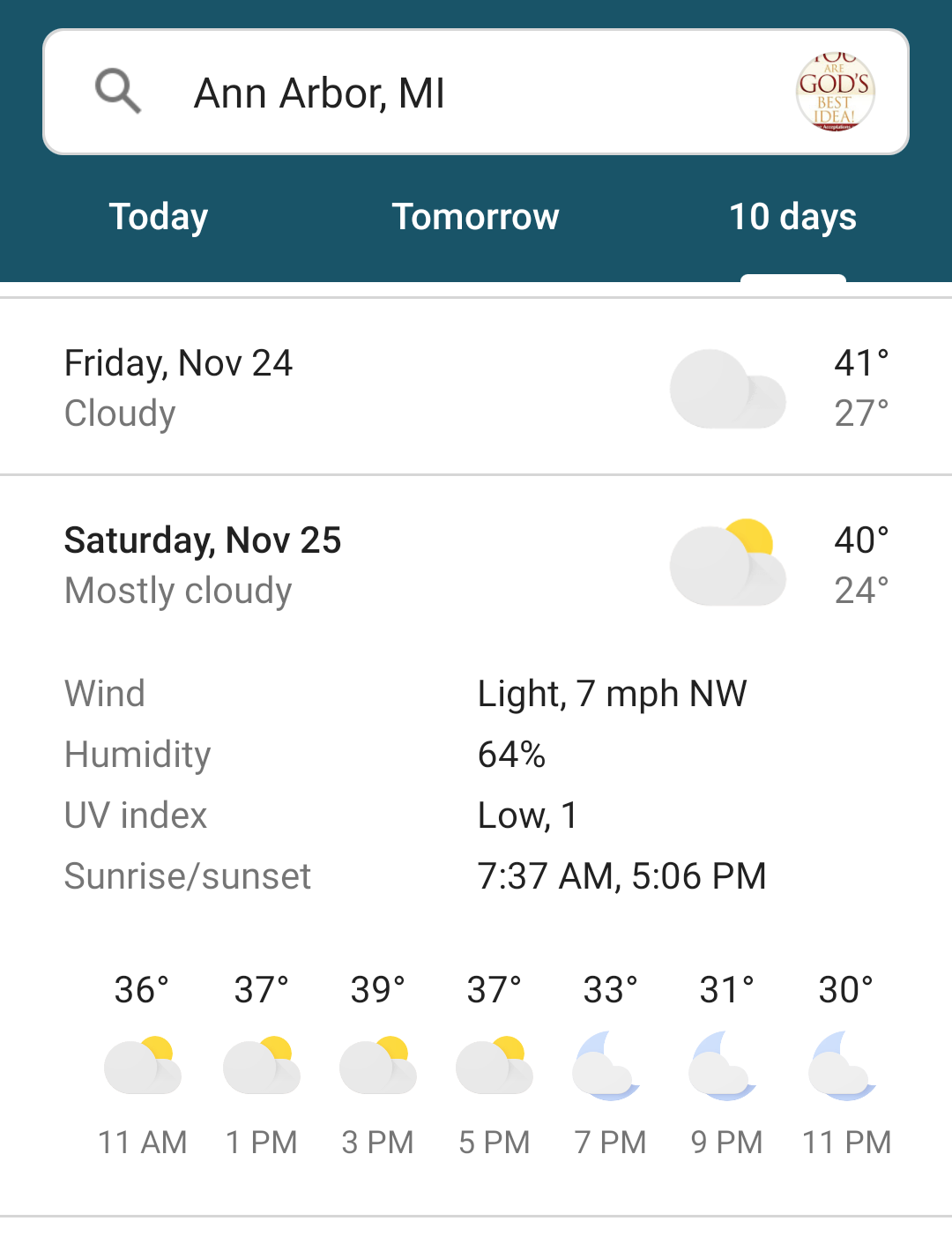Screenshot of a weather app displaying the forecast for Ann Arbor, Michigan. The interface shows a search bar at the top with "Ann Arbor, Michigan" entered. To the right, there is an ad partially cut off, reading, "to our God's best idea," enclosed in a circle.

The main forecast segment is set to "10 Days." Detailed weather information for Friday, November 24th, indicates cloudy conditions. An icon depicting a cloud is visible, alongside temperature highs of 41°F and lows of 27°F. Below, Saturday, November 25th, shows mostly cloudy weather with an icon featuring a cloud and a small sun behind it, suggesting partial sunlight. The temperatures for this day are a high of 40°F and a low of 24°F.

Additional weather metrics include:

- Wind: light, 7 mph from the northwest
- Humidity: 64%
- UV Index: low, 1
- Sunrise: 7:37 a.m.
- Sunset: 5:06 p.m.

Further, the hourly forecast displays time slots at 11 a.m., 1 p.m., 3 p.m., 5 p.m., 7 p.m., 9 p.m., and 11 p.m., with temperature readings as follows: 36°F, 37°F, 39°F, 37°F, 33°F, 31°F, and 30°F, respectively. Icons indicate mostly cloudy conditions transitioning to a different type of cloud icon suggesting nighttime.